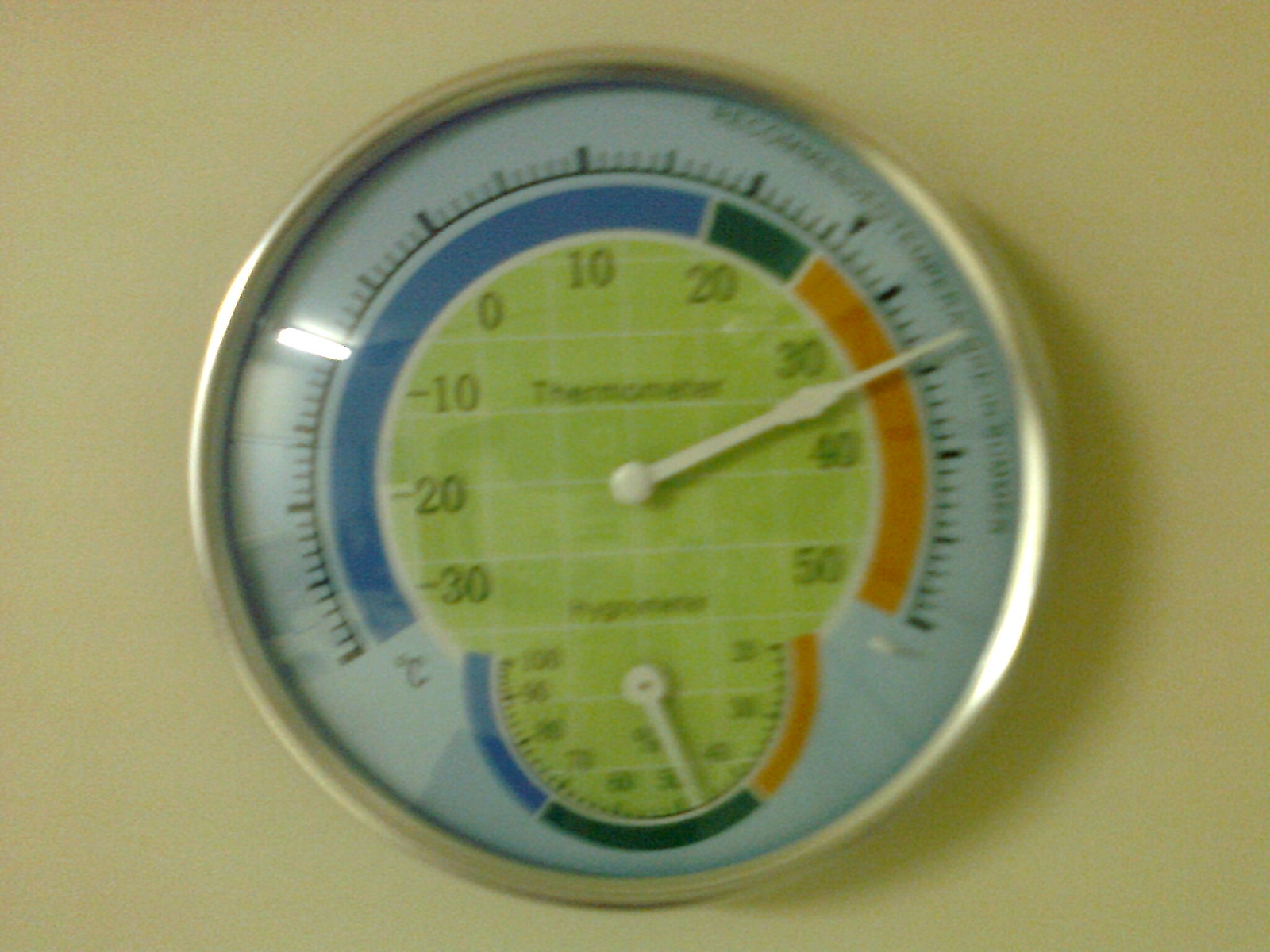The photograph depicts a thermometer set against a brownish backdrop, though the image is somewhat blurry. The central focus of the photograph is a circular thermometer encased in a silver metal border with a glass front. The internal design features a layered color scheme: the innermost section has a light blue background. Surrounding this, nearly completing a circle, is a dark blue arc extending slightly past the top middle. Adjacent to this is a narrow dark blue segment transitioning into a bright orange arc, which completes the semicircle.

Outside of this color band is a black line marked with small dashes circling the outer edge. The lime green interior of the circle displays text indicating "thermometer." Along the circle's periphery, numbers are denoted in a clockwise manner, starting from the left: -30, -20, -10, 0, 10, 20, 30, 40, and 50.

Beneath the main circle, there's a smaller, half-circle gauge that arcs in the opposite direction. This secondary scale is labeled with numbers in a counterclockwise order beginning from the left: 10, 90, 80, 70, 60, 50, 40, 30, and 20.